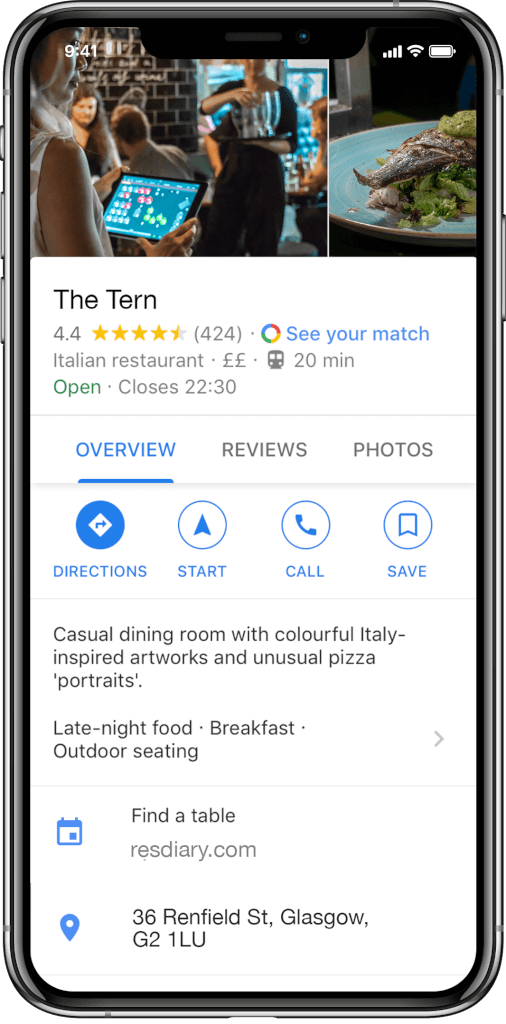A detailed screenshot of an iPhone display showcasing various elements. The iPhone has a grayish-black bezel with a button in the upper left and two larger ones beneath it, as well as a button on the right-hand side. The top center features the front camera lens area, with "9:41" displayed in white text. On the right, indicators show full cell signal strength, full Wi-Fi, and full battery.

The main content of the screen displays three images. The first image, on the left, captures a woman holding a tablet, seemingly engaged with a generic game, and looking away from others. The second, in the center, portrays a waitress in a black outfit carrying empty glasses on a serving tray in a restaurant setting. The third image, on the right, features a white plate with food, details of which are unclear.

Below the images, set against a white background in black text, "The Tavern" is prominently displayed. Next to this, in black text, it shows a rating of "4.4" accompanied by four and a half yellow stars and "424 reviews." A blue link reads "See Your Match." Underneath, in gray text, it specifies "Italian Restaurant" followed by two pound signs and an icon of a train with "20 min," indicating the distance.

Further details include a green indicator reading "Open" and in gray text, "Closes 22:30." Navigation options show "Overview" in blue with a line underneath, and "Reviews and Photos" in gray. Below are blue buttons labeled "Direction," "Start," "Call," and "Save."

A detailed description reads: "Casual Dining Room with Colorful Italian Inspired Artwares and Unusual Pizza Portraits, Late Night Food, Breakfast, Outdoor Seating," followed by an arrow pointing right. A calendar feature mentions "Find Your Table at rezdiary.com," and the address is listed as being in Glasgow.